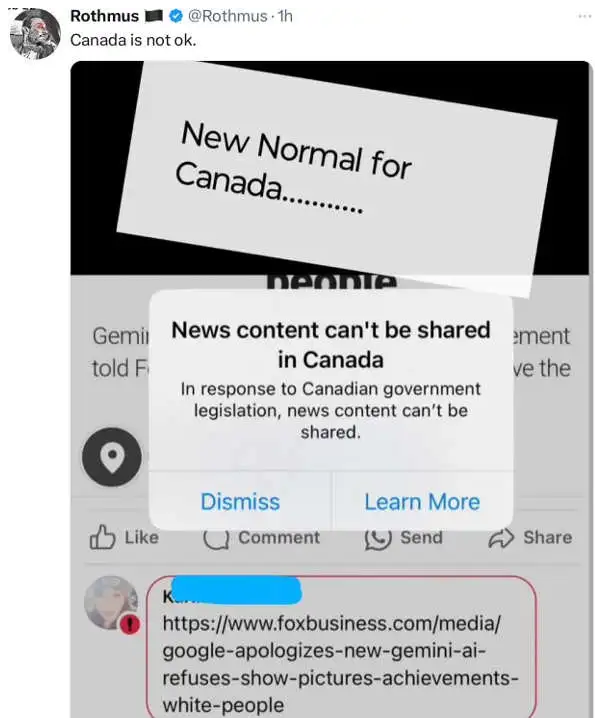The image showcases a social media post with a profile picture in the upper left corner labeled "Rothmus" and accompanied by the handle "@Rothmus" and a timestamp "1H". The main content of the post reads "Canada is not okay."

The main visual element of the image features a black rectangle at the top with a slightly off-center white rectangle over it, containing the text "New normal for Canada........."

Below this, a pop-up message is displayed, stating, "News content can't be shared in Canada. In response to Canadian government legislation, news content can't be shared." The pop-up offers two options in blue text: a "Dismiss" button and a "Learn more" link.

Towards the bottom, the image appears grayed out but contains a red-boxed URL: "http://www.foxbusiness.com/media/Google-apologizes-new-Gemini-AI-refuses-show-pictures-achievements-white-people."